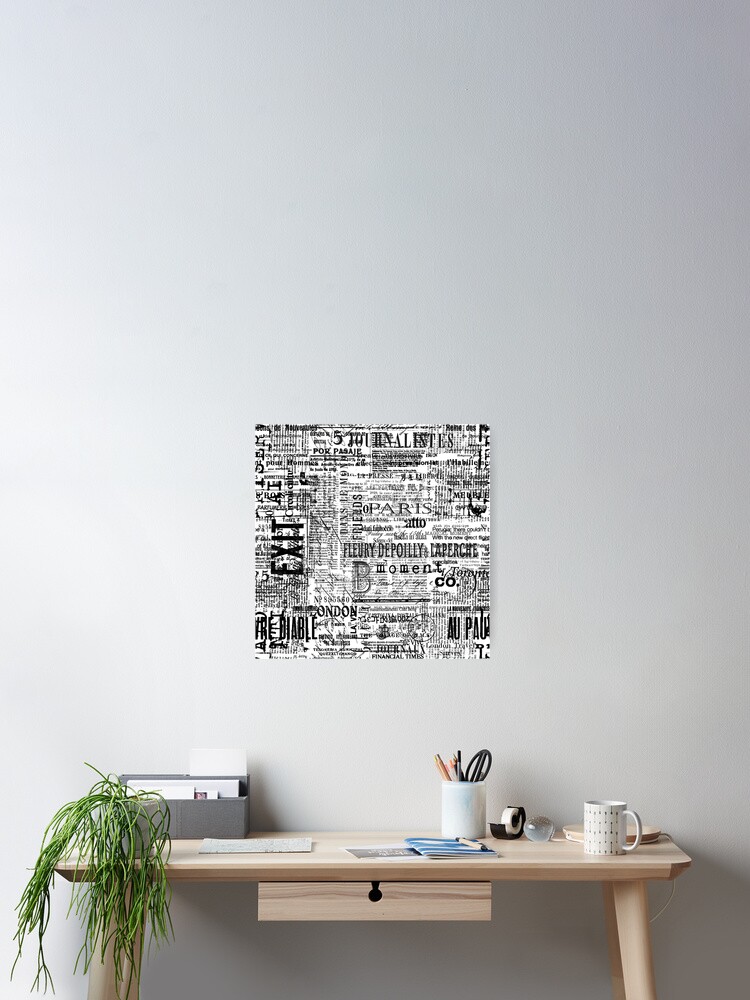The image depicts a minimalistic office setting featuring a small, light wooden desk with a single rectangular drawer beneath its tabletop, equipped with a little black slot resembling a keyhole. The desk is positioned against a plain white wall. To the left, a slightly wilted green spider plant resides alongside a gray desk organizer filled with papers or pamphlets. Dominating the wall above the desk is a square black and white poster showcasing various words in different fonts, with "exit" notably descending the left side. The right side of the desk houses a slender, white metal desk lamp with a 90-degree bend, sitting next to a distinct white coffee mug adorned with gold polka dots. Central to the desk's layout is another white cylindrical organizer brimming with pencils and scissors, accompanied by a black tape dispenser and scattered papers, including a closed magazine with a blue cover.